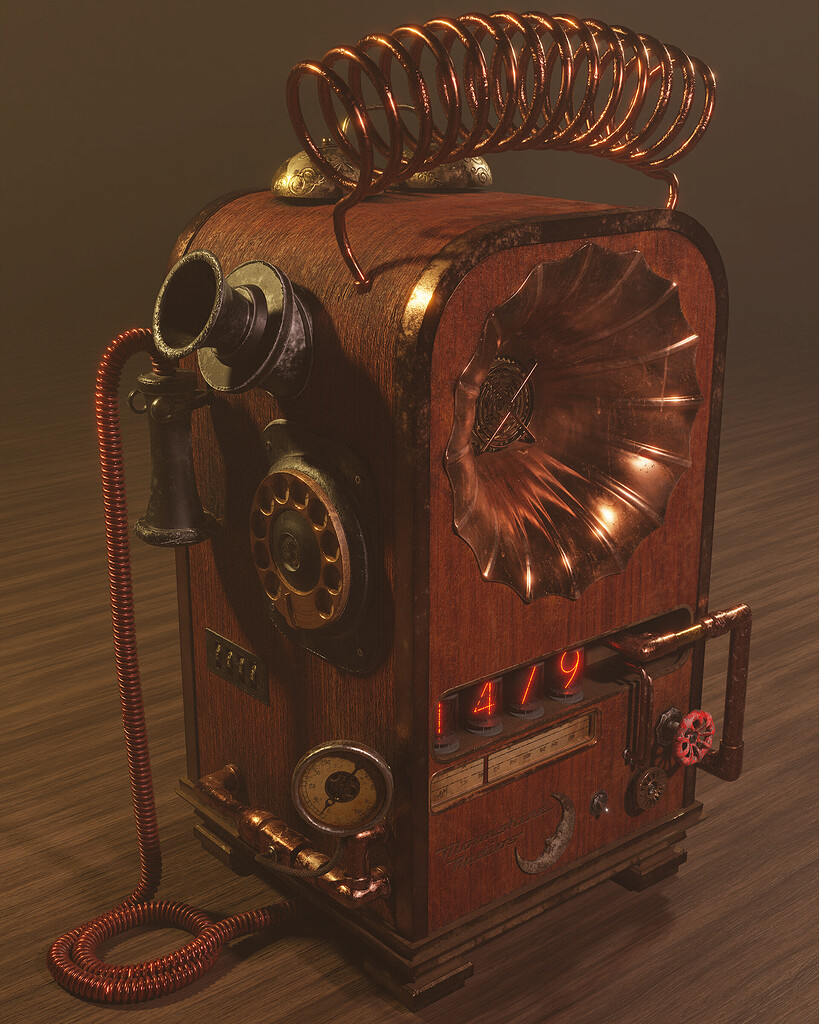This detailed photograph captures an intricate, vintage rotary phone housed within a large, square wooden box adorned with brass trim. The device features a rotary dial complete with numbers, a prominent pressure gauge at the bottom, and a substantial copper cord connecting the earpiece to the main body. Copper coils stretch over the top of the phone, adding to its complex appearance. Notably, the left side showcases a big speaker or horn-like structure, suggesting a possible gramophone functionality. The apparatus includes various elements such as valves and wires, with the top adorned by golden bells and a U-shaped copper coil. Adding to the intricacy, the machine displays the number "1479" at the bottom, hinting at it perhaps being a model within a steampunk-inspired setting. Overall, the object resembles a hybrid of antique telephone and early 20th-century machinery, evoking a multi-functional device from a bygone era.